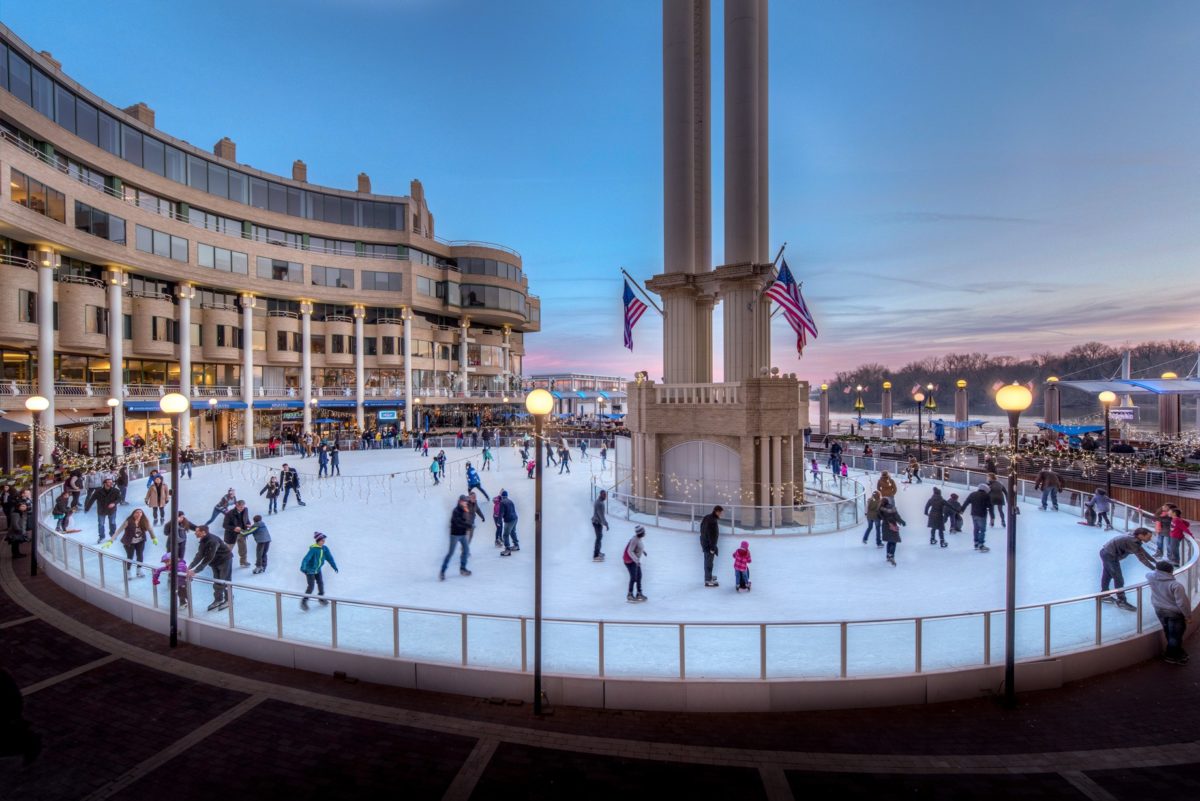The image captures a bustling circular ice skating rink set in a city center square during dusk. The sky exhibits a gradient from blue to the pinkish hues of a setting sun. At the center of the rink stands a tall column, extending out of the frame, adorned with at least three American flags. Surrounding this monument, skaters of all ages glide gracefully in a counterclockwise direction. The perimeter of the rink is lined with old-fashioned street lamps, casting a warm glow, and is enclosed by a short, see-through fence with glass panels. To the left of the rink, there is a large, pleasant-looking building, which could be a hotel or a shopping center, hinting at a cheerful atmosphere, likely part of a winter festival or a Christmas celebration.